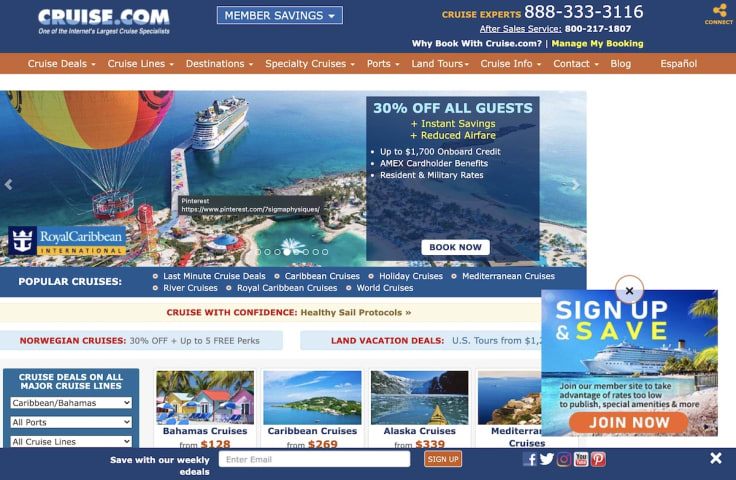The image showcases the homepage of the website cruise.com, prominently featuring their branding and a slogan, "One of the internet's largest cruise specialists," at the top. The upper right corner of the page includes a contact section labeled "Cruise Experts" with the phone number 888-333-3116. Just below this header, an orange navigation banner organizes key website sections: Cruise Deals, Cruise Lines, Destinations, Specialty Cruises, Ports, Land Tours, Cruise Info, Contact Blog, and Español.

Central to the page is a large, eye-catching image depicting a picturesque harbor scene, likely representing a potential cruise destination. This tropical setting includes clear, blue waters, a majestic cruise ship, a hot air balloon, and attractions reminiscent of rides and theme parks. 

On the bottom left of the image, there is a promotional box for Royal Caribbean International, offering special deals such as 30% off for all guests, instant savings, reduced airfare, up to $1,700 in onboard credit, Amex cardholder benefits, and special rates for residents and military personnel. Adjacent to this offer is a prominent "Book Now" button in white.

Below the image, the page highlights a list of popular cruise categories including Last-Minute Cruise Deals, Caribbean Cruises, Holiday Cruises, Mediterranean Cruises, River Cruises, Royal Caribbean Cruises, and World Cruises. 

Further down, a yellow banner with the phrase "Cruise with Confidence" is displayed before listing various cruise options along with their respective prices.